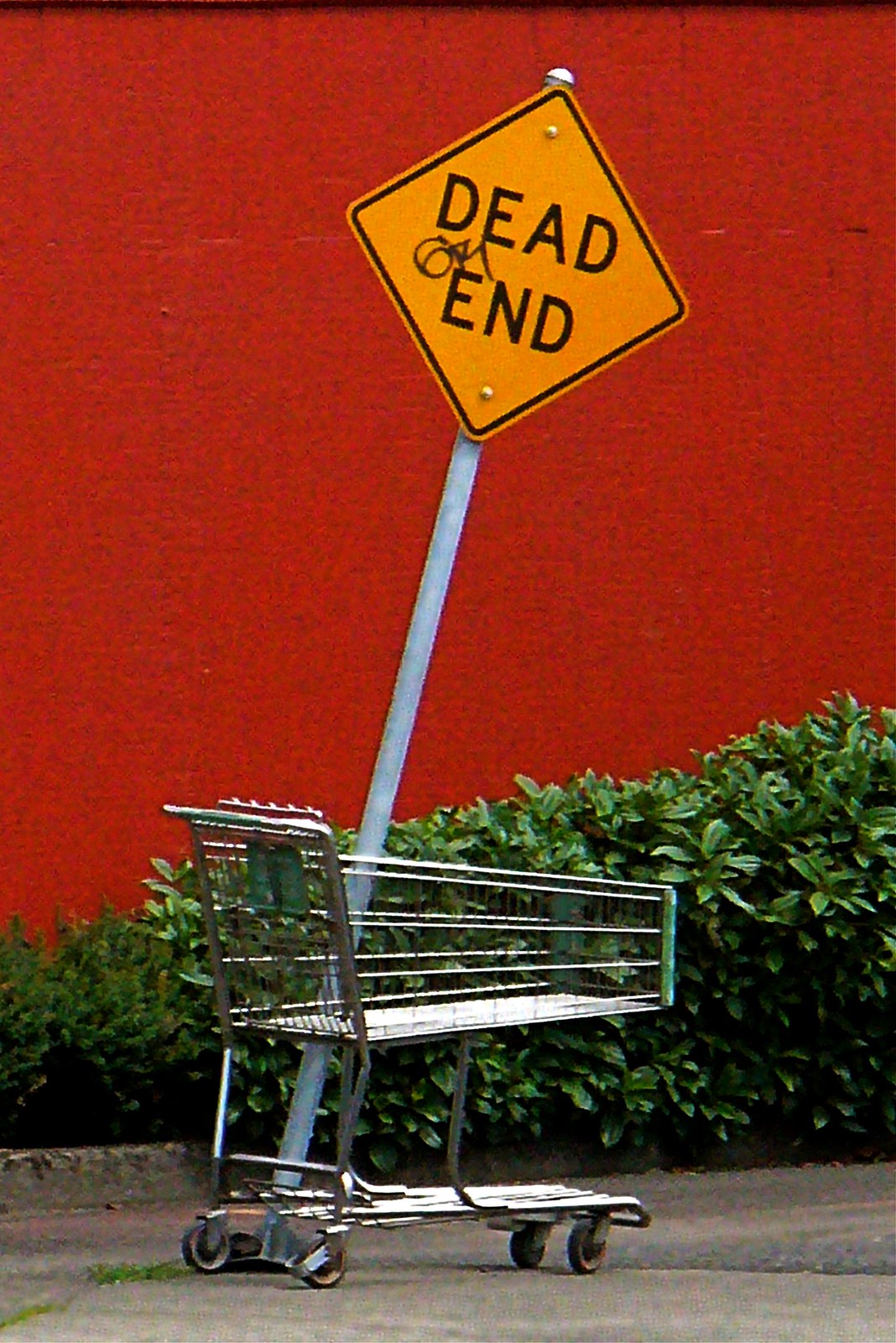This outdoor photograph features a predominantly red wall occupying the top three-quarters of the image. Below the wall, a vibrant green shrub and several bushes add a natural element against the stark backdrop. At the bottom, a gray concrete surface extends across the frame. Positioned left of center at the bottom, a gray pole tilted to the right rises from the concrete. Atop the pole, a triangular yellow sign with a black outline and bold black text reads "DEAD END," with some graffiti markings scribbled above the letter 'E'. In front of the pole stands a silver metal grocery cart, viewed from its right side, with the handle visible on the left. The cart has a bottom platform and a distinctive green strip along the front edge, completing this urban scene.